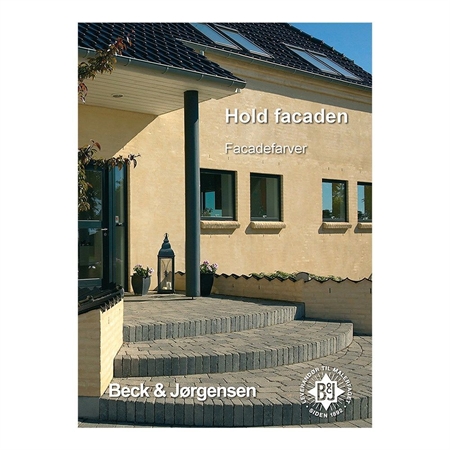The image showcases a newly constructed, light tan building, possibly commercial, with a clean and organized exterior. The building features a medium-sloped black roof with what appear to be small windows or skylights, possibly solar panels. Along the side, there are several large windows. The front door, reminiscent of a business entrance, is reached via three gray and tan brick risers and is flanked by a decorative planter and a large black lantern. An overhanging awning supported by a single pole casts a shadow, indicating sunny weather. The image includes partial text and a logo from Beck and Jorgensen, suggesting this could be an architectural or exterior design demonstration. The text reads "Hold Fakaden, Fakade Farver," and appears in another language. The scene is accented by various shades of tan, yellow, black, and gray, with a bit of a tree peeking from the left side, providing a touch of greenery.